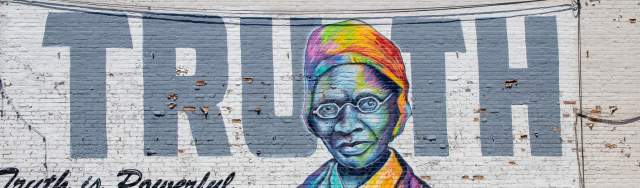The image features a wide and thin mural painted on the white-brick siding of a building. A black wire runs across the top of the mural and descends along the right side. Dominating the mural is the vibrant depiction of a black woman with full lips, high cheekbones, a wide nose, and small, almost oval wire-framed glasses. She is adorned in a colorful head wrap with hues of purple, green, blue, yellow, red, and orange, and a collared shirt in shades of blue, orange, and purple. Her face features an intriguing blend of bluish tones with purple highlights. The background showcases large, steel-blue block letters spelling out “TRUTH,” and in the bottom left corner, the phrase “TRUTH IS POWERFUL” is visible in black, although parts are partially cut off in the image.